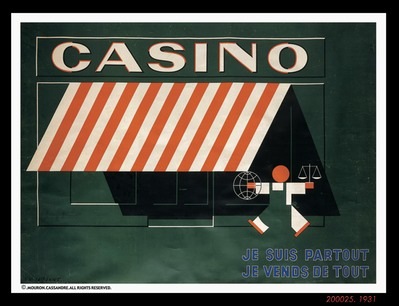The image features a sketched, animated storefront with artistic detailing, encapsulated within thin black and white frames. Dominating the sign above the storefront is the word "Casino" in large white block letters outlined in orange and black, set against a very dark green background. Beneath "Casino", an orange and white striped awning stretches downward, partially covering a doorway with windows. To the right, under the awning, stands a simplistic stick-figure man characterized by an orange head devoid of facial features, adorned in white clothes and an orange apron. In his hands, he holds a white scale and an outlined globe. Intricate details such as his white shirt, white pants, and orange shoes add to his distinct appearance. The lower right corner of the green storefront background bears French writing, "Je suis partout, je vends de tout," indicating "I am everywhere, I sell everything." Additionally, there are numbers inscribed: 20002.5.1931, and a note on the bottom left states, "All rights reserved." The overall main color scheme is dark green, accentuated by details in orange, white, and black.